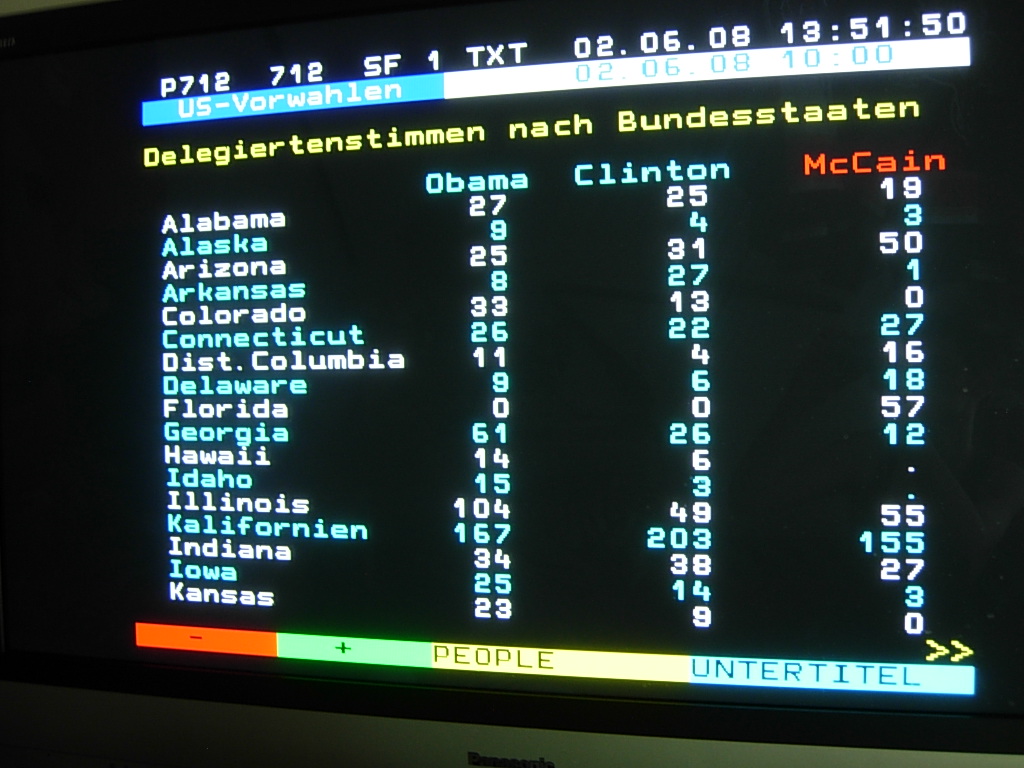The image is a rectangular photograph of a Teletext screen displaying the 2008 US primary election results, reportedly from a system in Switzerland. The screen has a black background with digital text and numbers spread across it. At the top of the screen, there are blue and white bars showing the date and time, followed by some text in a foreign language. Below this, the screen is divided into four main columns. The leftmost column lists the US states from Alabama to Kansas. The next three columns display the results for the candidates Obama, Clinton, and McCain, with Obama’s and Clinton’s numbers in blue, and McCain’s in red. Each state’s corresponding results are numerically listed in these columns; for example, Alabama shows Obama with 27, Clinton with 25, and McCain with 19 votes. Towards the bottom of the screen, there is a bar in orange with a minus sign, followed by green with a plus sign, and the labels "people" and "uter-title" in yellow and blue, respectively.